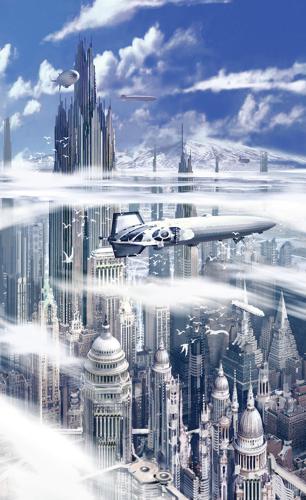The digital artwork depicts a futuristic cityscape viewed from above, featuring an array of skyscrapers piercing through a blanket of white clouds. Dominating the skyline are numerous tall buildings with dome-shaped tops, reminiscent of the US Capitol building, interspersed with other architectural designs including pyramid and pointed tops. The urban scene is predominantly rendered in shades of white and gray, enhancing its sci-fi aesthetic.

In the center right of the image, a sleek, white airship with blue trim and windowed details gracefully floats amidst the towering structures. Meanwhile, a pair of smaller blimps can be seen near an exceptionally tall skyscraper on the left side of the image, their delicate forms contrasting against the imposing architecture. The sky above is alive with activity, as flocks of white birds soar freely, contributing to the dynamic atmosphere of the scene.

Framing the city in the distance, a mountain range with snow-capped peaks rises majestically, further enriching the composition. The bright blue sky and thick clouds in the background complete this breathtaking vision of a futuristic urban utopia, where advanced technology seamlessly integrates with natural beauty.